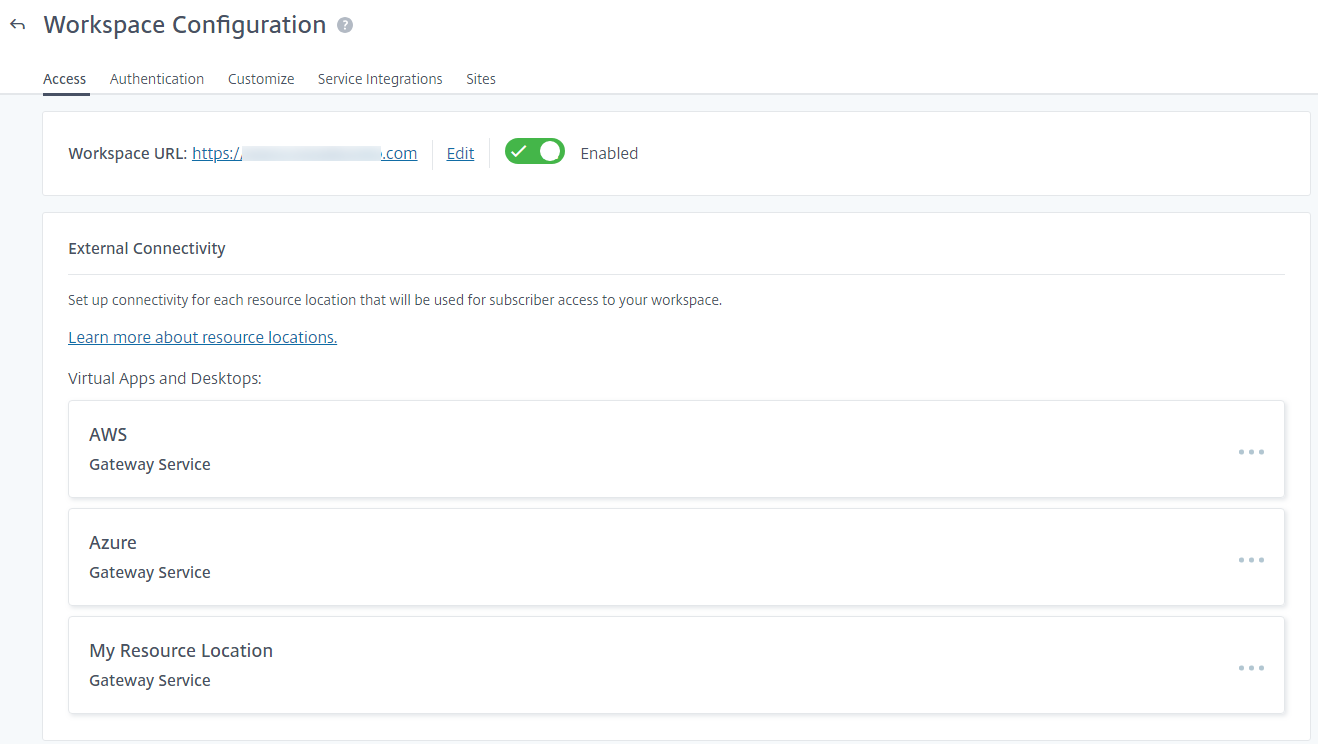**Detailed Workspace Configuration Screenshot Caption:**

The image showcases a detailed workspace configuration interface on a computer. The top left corner features the title "Workspace Configuration" in bold black font. Directly beneath the title, there are five categorized drop-down menus: "Access," "Authentication," "Customize," "Service Integration," and "Sites." The currently selected category is "Access," highlighted to differentiate it from the others. Below these menus, a light blue or gray box displays the configurations available within the "Access" category. The user has enabled and defined a specific workspace URL, ensuring it allows access. Further settings include managing overall external connectivity by selecting various virtual applications and desktop environments. Notably, AWS and Azure, along with other similar services, are listed as accessible options, emphasizing the comprehensive setup for external service integration.